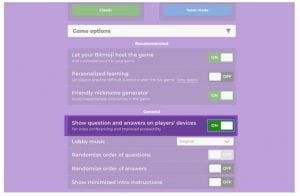The image depicts a website interface with a predominantly white background. At the top of the page, there are two colored patterns: the one on the top left is green, and the one on the top right is blue. The text on the website appears blurry and unreadable, compromising its visibility.

Beneath these two patterns, there is a drop-down option labeled "Common Options" in black text. Accompanying this drop-down menu, an error message indicates that there is an issue with selecting an option. Below this section, several toggle switches are arranged in sequence. 

The first toggle switch is turned on, displaying a green color. The second toggle switch is turned off and appears grey. The third toggle switch is also on and green. While the switches that are on display a green hue, the visibility of the accompanying text is compromised for the grey (off) switch. 

Towards the bottom part, an additional toggle switch is in the on position with a green indicator. Alongside this, there is a list containing three options, all of which are off. 

Lastly, the entire page's background transitions into a gradient of purple and green, with toggle switches in their respective colors of green for "on" and grey for "off." The text throughout the page is predominantly written in white, except for the "Common Options" text, which is in black. The overall presentation suggests a colorful but somewhat dysfunctional interface due to the blurriness and unreadable text.